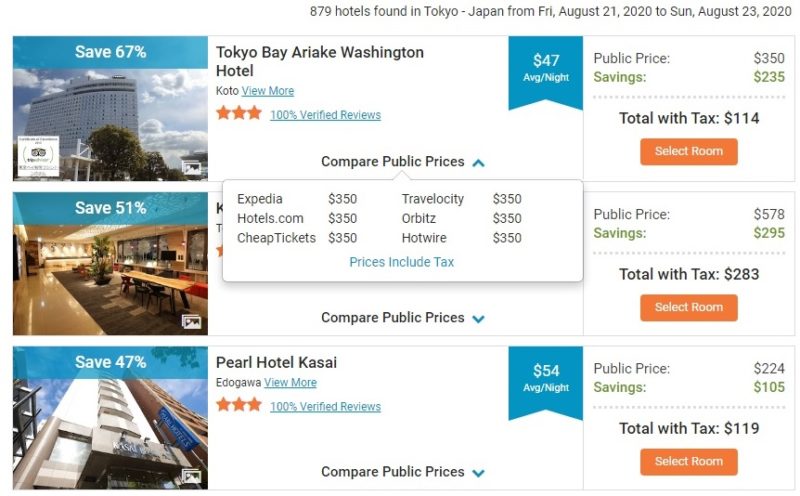**Detailed Descriptive Caption:**

This screenshot displays booking information for various hotels in Tokyo, Japan, scheduled from Friday, August 21st, 2020, to Sunday, August 23rd, 2020. The background is white with dark gray text at the top right corner, indicating that 879 hotels were found in Tokyo for the mentioned dates. There are three rows showcasing different hotels with accompanying details.

**First Row:**
- On the left side is an image of the Tokyo Bay Ariake Washington Hotel, featuring a white building against a blue sky with clouds. A green rectangle overlays the image with white text that reads "Save 67%."
- To the right of the image, the hotel's name is displayed in black font followed by the location "Koto" in a smaller font. 
- Below the name are three orange stars, denoting the hotel's rating, and a blue text link reading "100% verified reviews."
- Adjacent to this information is a blue ribbon-shaped icon with "$47 average per night" text.
- A drop-down menu below this section allows for price comparison among various booking platforms including Expedia, Hotels.com, CheapTickets, Travelocity, Orbitz, and Hotwire. All listed prices include tax and amount to $350.
- Further to the right, cost information highlights the top public price as $350 with a green-saving annotation showing $235, resulting in a total of $114 with tax included.
- An orange rectangle at the far right with white text offers an option to "Select Room."

**Second Row:**
- The image shows an interior view of a hotel lobby with a green overlay text indicating "Save 51%."

**Third Row:**
- The image depicts a hotel viewed from the bottom looking upwards and features a similar green overlay text reading "Save 45%."
- Text next to the image identifies the hotel as Pearl Hotel Kassai, followed by additional price and booking details.

Each row provides a comprehensive overview of the hotel options, prices, savings, and booking links available for prospective travelers.